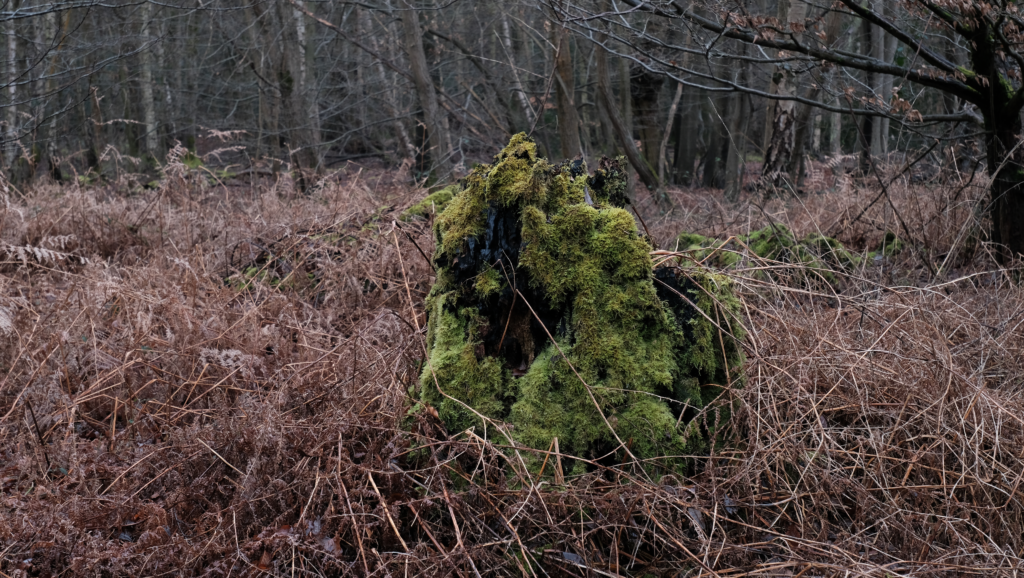In the center of this forest scene stands a large, green moss-covered structure, with hues of light green mixed with patches of brown. This mossy formation is nestled among a predominantly light brown landscape filled with dead grass and dried-out brush, suggesting it is either late fall or winter. Surrounding the structure, the background is populated by tall, thin tree trunks that are mostly grayish-brown and devoid of leaves, adding to the somber seasonal atmosphere. Notably, there is a bare tree close to the right of the mossy structure, extending long, black branches across the middle of the image. The peculiar shape of the moss suggests various interpretations; some see it as a camouflaged hunting hut with an opening at the front, while others describe it as resembling a wide, gorilla-like figure with arm-like extensions and a short back. This blend of natural elements creates an intriguing and mysterious woodland scene.